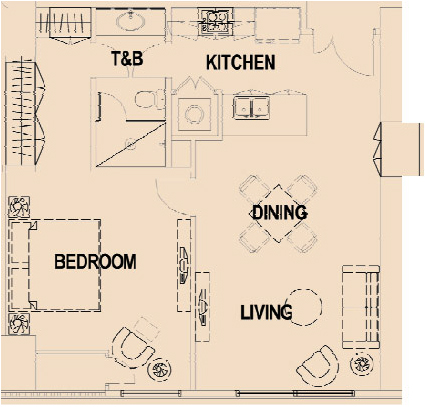The sketch depicts a detailed floor plan of a potential apartment. The entrance doors lead directly into a dining room, which is furnished with a table and four chairs. Adjacent to the dining room is the kitchen, equipped with a sink, stove, refrigerator, and possibly a closet or pantry. Below the dining room is a cozy living room area, complete with a couch, armchair, coffee table, and a side table. The dining room seamlessly connects to this space.

To the left of the kitchen and at the top of the illustration, labeled "T and B," is a bathroom featuring a sink, toilet, and shower. Built-in bookshelves appear to be integrated into the walls. Below the bathroom, there is a bedroom furnished with a double bed, a dresser with a TV on top, a chair, and a side table. The overall layout suggests a compact but efficiently designed apartment.